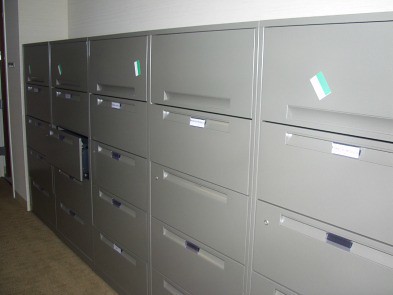This is a detailed color photograph of a wall lined with five file cabinets, each featuring five rows of light gray metal drawers, totaling almost 25 compartments. Labels adorn some of these drawers, including white labels and distinctive rectangular stickers that are half white and half turquoise blue. One drawer, specifically in the second column and third row from the top left, is slightly open, revealing a black interior but no visible contents. The cabinets align against a white wall, with a light brown tan carpet extending across the floor at the base. Each drawer has an indentation near its bottom for easy opening, and various labels and sticker arrangements are evident on these drawers.